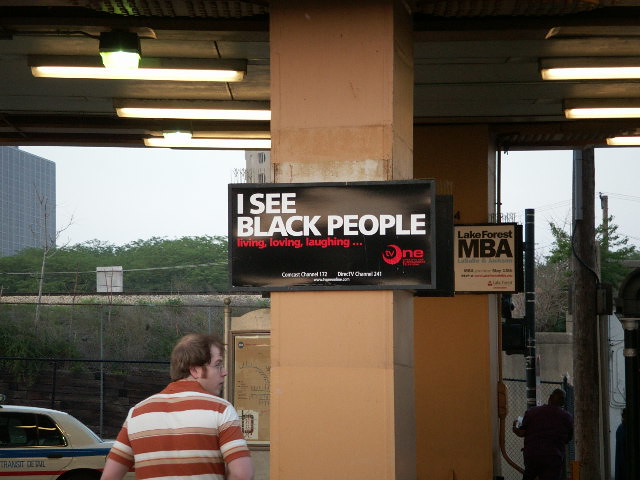In the foreground of the urban street scene, a prominent concrete pillar stands as a central element. This square pillar is adorned with a black sign featuring bold text: "I see black people" in white lettering, and "living, loving, and laughing" in red. Beneath this, the sign reads "Lake Forest NBA."

The background reveals elements of urban greenery, with bushes and possibly trees, blending into the distant cityscape under a clear sky. Hints of buildings peek through the vegetation.

On the left side of the image, a white male with his back to the camera, dressed in an orange and white striped shirt, gazes to the right. A transit car, partially visible in the bottom left corner, suggests movement or a bustling environment.

To the right, another figure can be seen from behind, wearing dark clothing. This person appears to be entering a fenced area, adding a layer of depth and narrative to the scene.